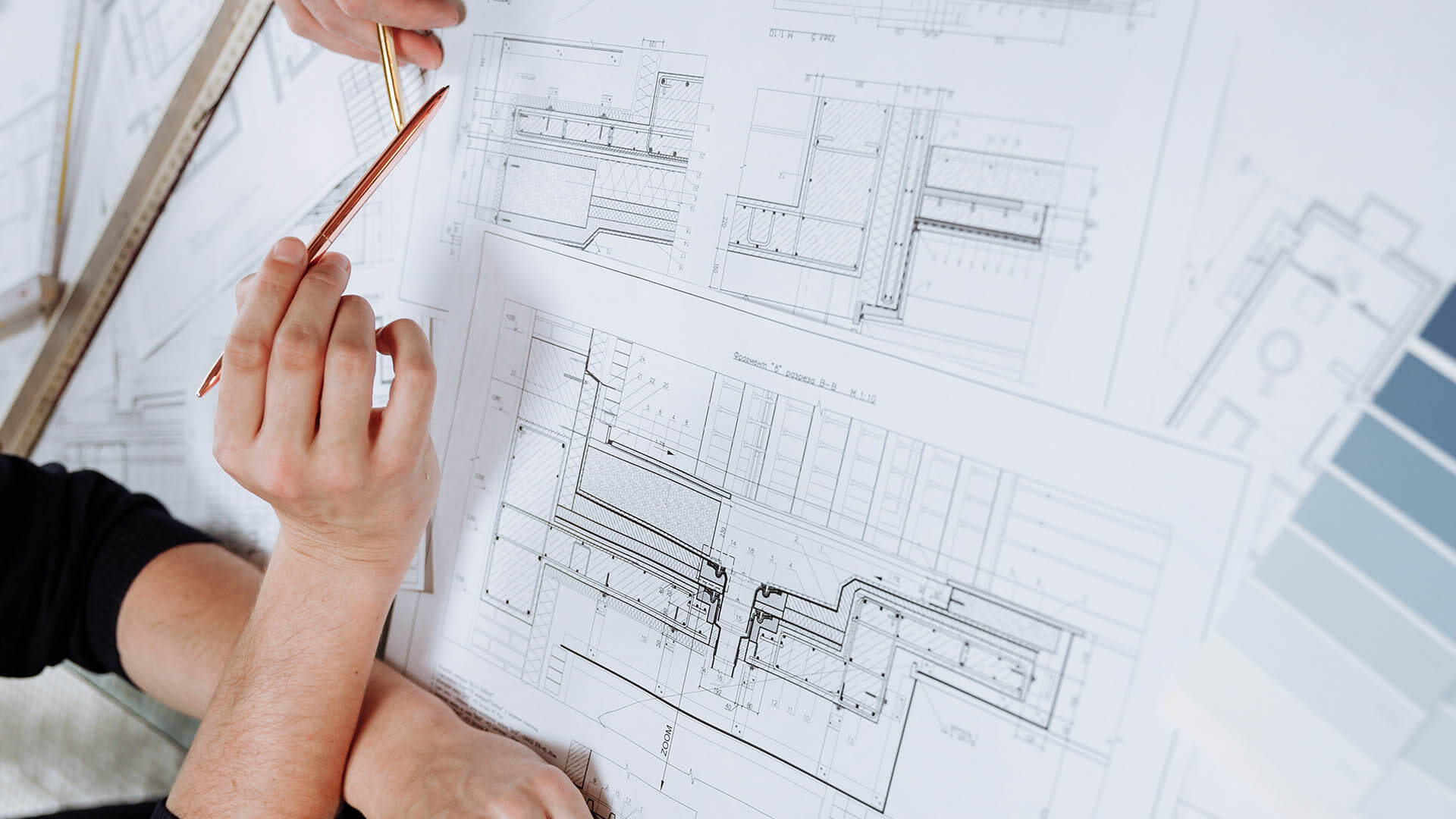The image features a detailed scene of two individuals examining architectural plans. The plans, primarily white with black schematics, occupy most of the table's surface. One individual, dressed in a long-sleeved black shirt, has their hands crossed on the left side of the image; one hand grips a gold pen while the other rests on the table. The second person's right hand, partially visible at the top of the image, also holds a gold ink pen. A large silver ruler and a protractor-like tool are positioned across the drawings.

The architectural plans are meticulously detailed and appear to be schematics for ductwork or electrical systems, though the specific labels on the plans are too small to read. The scene is infused with tones of muted blues, highlighted by a paint chip in the lower right corner, showcasing a color palette. The two individuals seem to be focused on a particular section of the plans, underscoring a collaborative effort in their review and discussion.